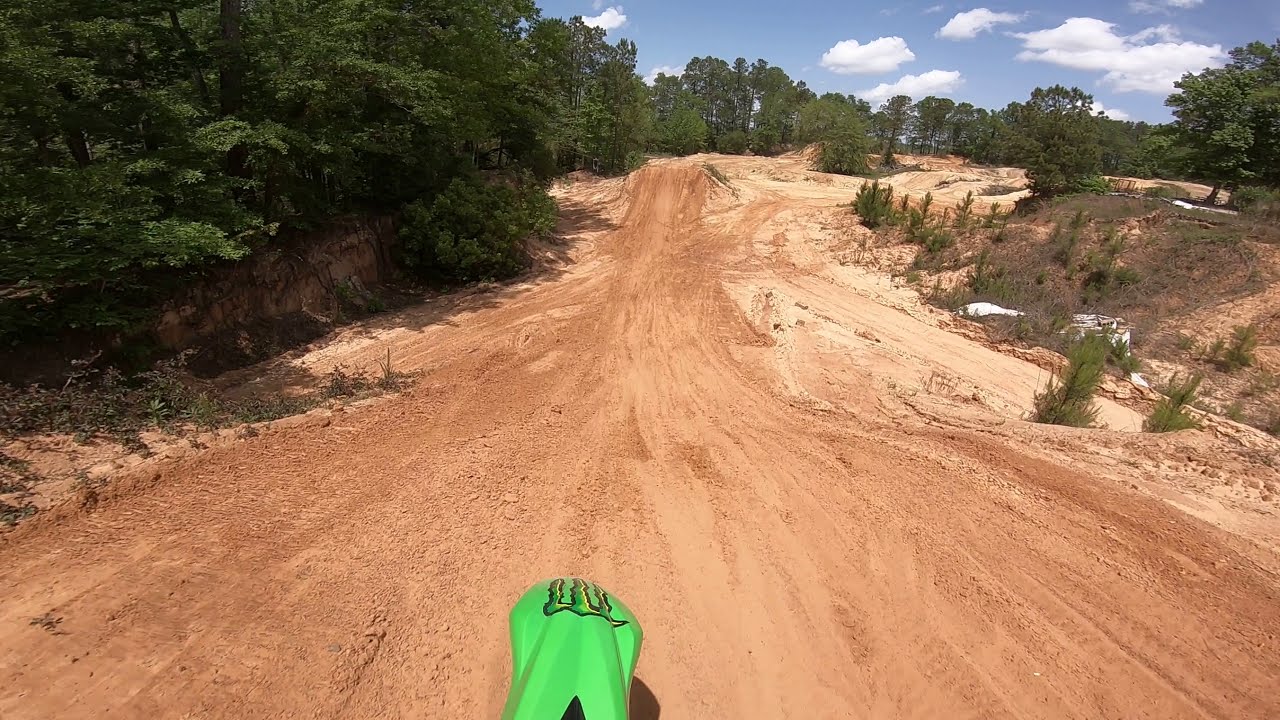This photograph captures an uneven dirt road covered in brown soil, extending from the bottom and narrowing towards the horizon. The image is taken from the perspective of someone on a green motorbike, with the bike's green metallic tire cover and a distinct logo visible at the bottom center. To the left of the road, a dense forest of lush, dark green trees continues into the distance. On the right, the landscape features small green plants, dried vegetation, and a lighter dirt path intersecting the main road further down. Some sporadic pine trees and a slightly sloping terrain add to the scene's depth. The sky above is a vibrant blue, adorned with wispy white clouds, framing the natural setting beautifully.